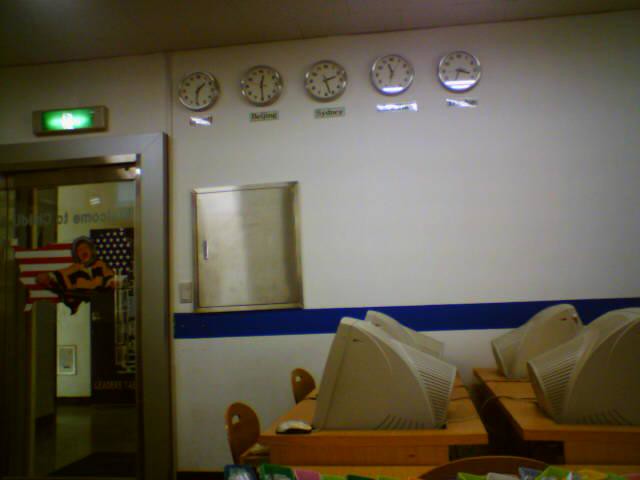The photograph captures an interior shot of a room that appears to be a computer room, potentially within a US government office, based on the presence of a painted or decal flag on a door. The room has an older, somewhat outdated appearance, likely pointing to it being taken around 15 to 20 years ago. The central focus involves two rows of brown wooden desks each equipped with sizable, boxy, white computers reminiscent of those from the 1990s or early 2000s. 

On the right-hand side of the room, there are three desks on either side, totaling six desks. Atop these desks are older computer monitors, and some have wooden chairs placed on them. The back wall, which is white, is accentuated by a thick blue horizontal stripe. Above this stripe, there is a small silver door, possibly for maintenance or storage, and a standard door adorned with a painted or decal US flag and the image of a woman. This door also has a green exit sign above it.

Dominating the upper portion of the back wall are five prominently displayed clocks with white faces, black numerals and hands, and silver trim, each showing different times, suggesting various global time zones such as Beijing and Sydney. The names of these time zones, though blurred, are inscribed below each clock. Near the door, there's a silver metallic fixture attached to the wall, which has a green light above it, further emphasizing the official, possibly governmental nature of the room.